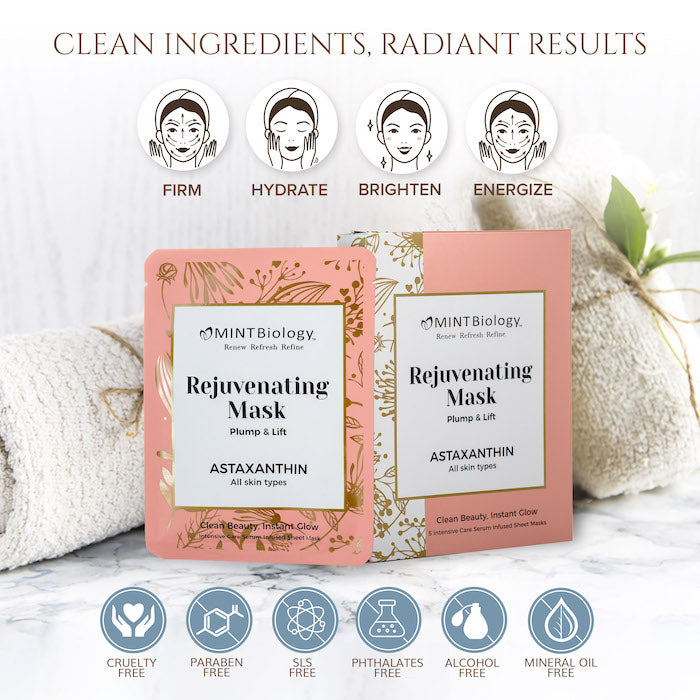The advertisement showcases a rejuvenating face mask from Mint Biology. At the top of the image, bold text reads "Clean Ingredients, Radiant Results." Below this, there are four panels featuring the same woman applying the mask, each labeled with different benefits: Firm, Hydrate, Brighten, and Energize. The central part of the image highlights the product's packaging—a pink container with golden accents and curving vines. The text on the package includes "Mint Biology" and "Rejuvenating Mask - Plump and Lift," with "Astaxanthin, All Skin Types" specified beneath. The product is framed by pillows on both sides. Further down, circular icons in dark blue detail that the mask is cruelty-free, paraben-free, SLS-free, phthalate-free, alcohol-free, and mineral oil-free.